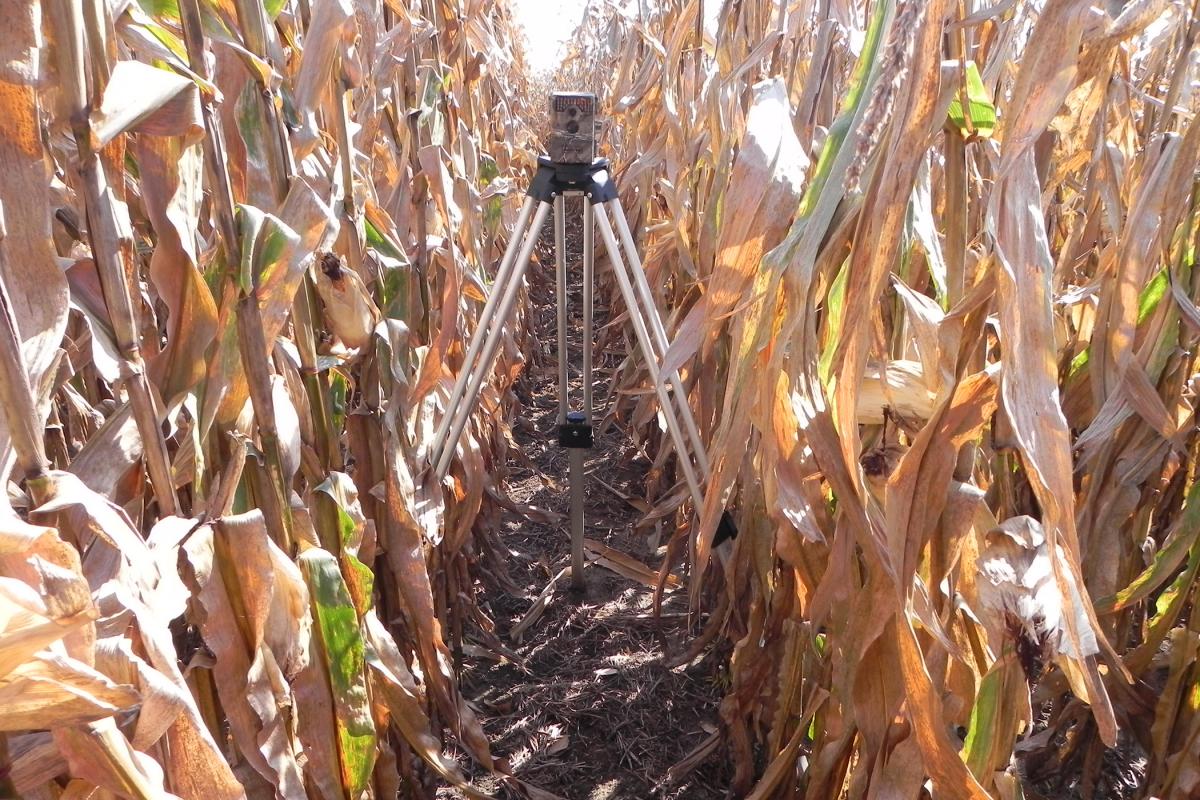In this photograph, taken in landscape orientation in what appears to be a cornfield, the scene is set during the autumn or early winter months. The corn stalks, visible in long, dense rows stretching out to the horizon, are predominantly dried, shriveled, and brown with only sporadic hints of green. The dried husks seem brittle, as though they might crumble at the slightest touch. In the center of the image, positioned in a narrow pathway between the rows of corn, stands a tripod with silver legs. Atop the tripod is a rectangular, camouflage-patterned device resembling a game trail camera. This device, equipped with a viewfinder and lens-like components, suggests it's used for surveying the land or monitoring wildlife activity. The tripod and camera form the focal point against the backdrop of the vast and desolate-looking cornfield, emphasizing the season's end and the landscape's stark, rustic beauty.